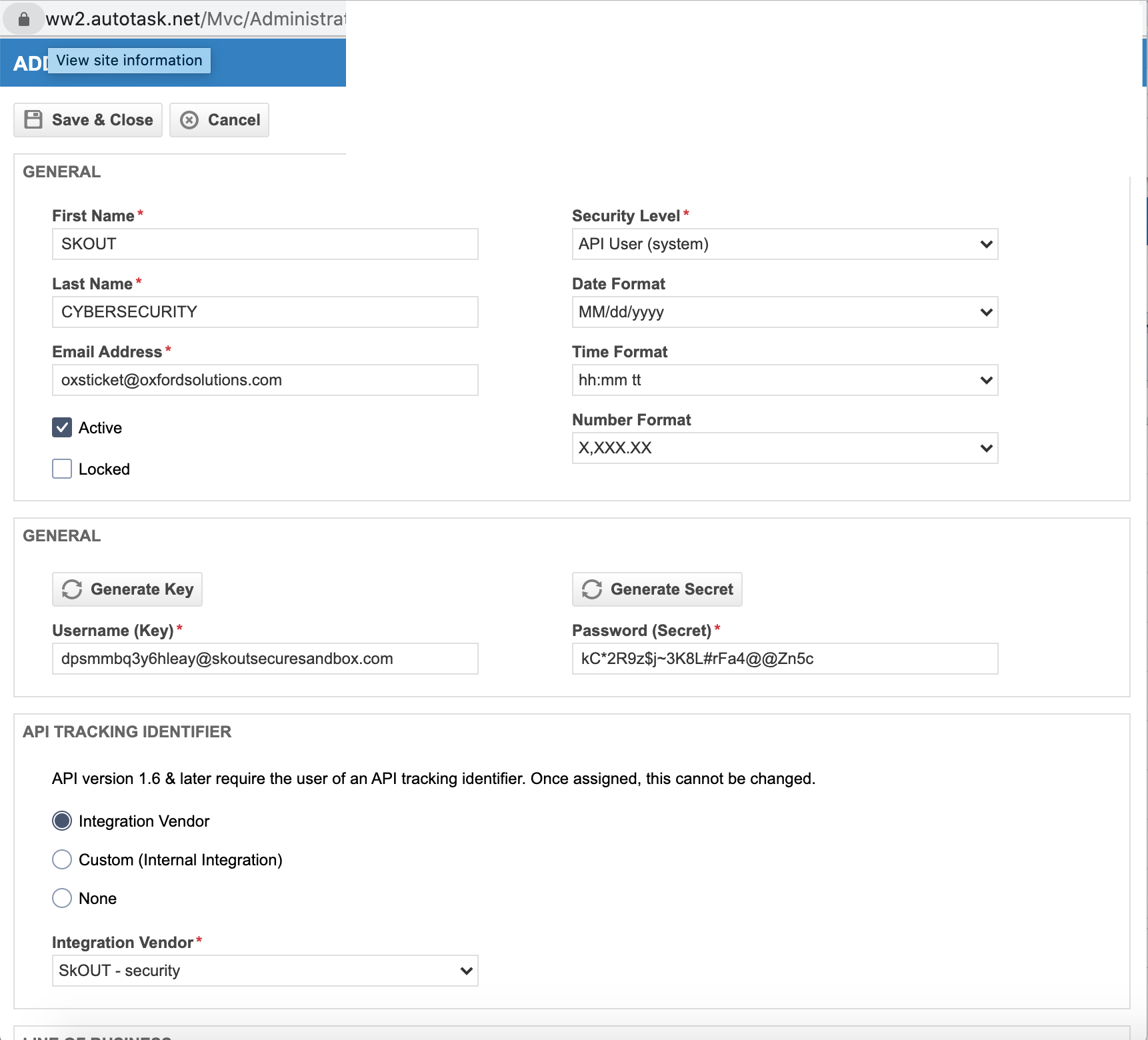The image features a user interface with a predominantly gray outline, although on the right-hand side, the outline is only partial. At the top, there is a light gray rectangle housing a slightly darker gray oval with a lock icon inside. Adjacent to this is a section labeled with a website. Below, a dark blue rectangle partially displays the letters "AD," obscured by a lighter blue rectangle bearing the text "View Site Information."

Further down on the left, a gray rectangle contains the words “Save and Close,” accompanied by a disc icon. Next to it, a light gray rectangle with a circle and an “X” holds the word “Cancel.” The section below is titled "General," followed by fields for "First Name" and "Last Name" with gray outlined rectangles. Both fields have red stars indicating required input.

Below these, there are fields labeled "Email Address" and "Security Level," each accompanied by gray outlined rectangles. The "Security Level" field is populated with "API User System" and features a downward arrow. In subsequent sections, labels for "Data Format," "Time Format," and "Number Format" are each paired with gray outlined rectangles and downward arrows. 

On the left, another "General" section includes gray rectangles for "Generate Key" and "Generate Secret," each with a circle and two arrows icon. The section continues with labels for "Username (Key)" and "Password (Secret)," each with gray outlined rectangles containing placeholder text, both marked with red stars and followed by text boxes with respective content.

There is also an "API Tracking Identifier" field, followed by "API Version" in smaller text. Below, a blue circle marked "Integrate" is present, with adjacent gray circles labeled "Custom (Internal Integration)" and "None." Another section labeled "Integration Vendor" also includes a gray outlined circle for "Scout Security" with a downward arrow.

The comprehensive layout captures each field and element, illustrating the organization and functionalities within this particular user interface.